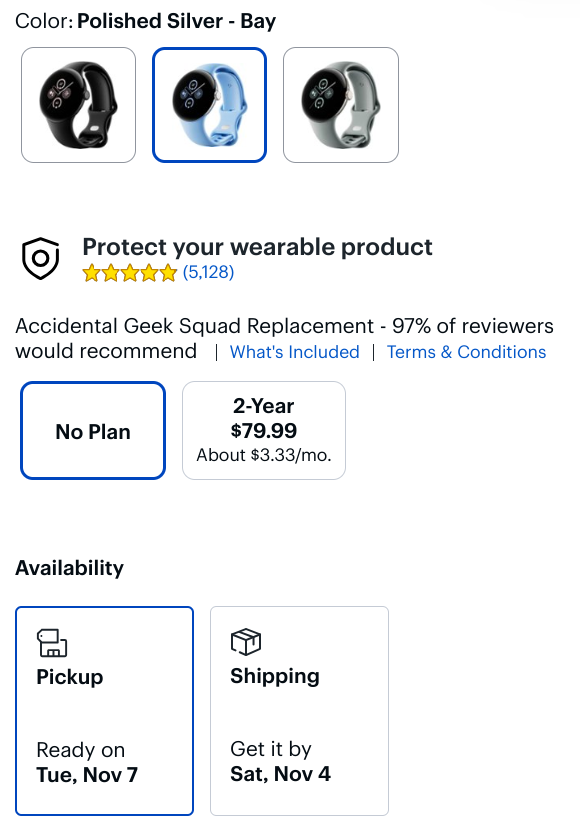Here's a polished and detailed caption for the image described:

---

The shopping page features a sleek, polished silver smartwatch on a white background. At the top, the "Color: Polished Silver" label appears in bold black text. Below, three square thumbnails display different watch models, with the middle option highlighted by a distinct blue border. This selected model showcases a light blue band paired with a black round face.

Further down, a "Protect Your Wearable Product" section boasts an impressive five-star rating from 5,128 reviews. Beneath this, the option for "Accidental Geek Squad Replacement" is noted, highlighting that 97% of reviewers would recommend this protection plan. Shoppers can choose between "No Plan" or a "Two-Year Plan" priced at $79.99, which breaks down to about $3.33 per month.

In the "Availability" section, customers can select either "Pickup" or "Shipping." The current selection is "Pickup," with an estimated readiness date of Tuesday, November 7th.

---

This caption offers a comprehensive and organized description of the product webpage's features and options.